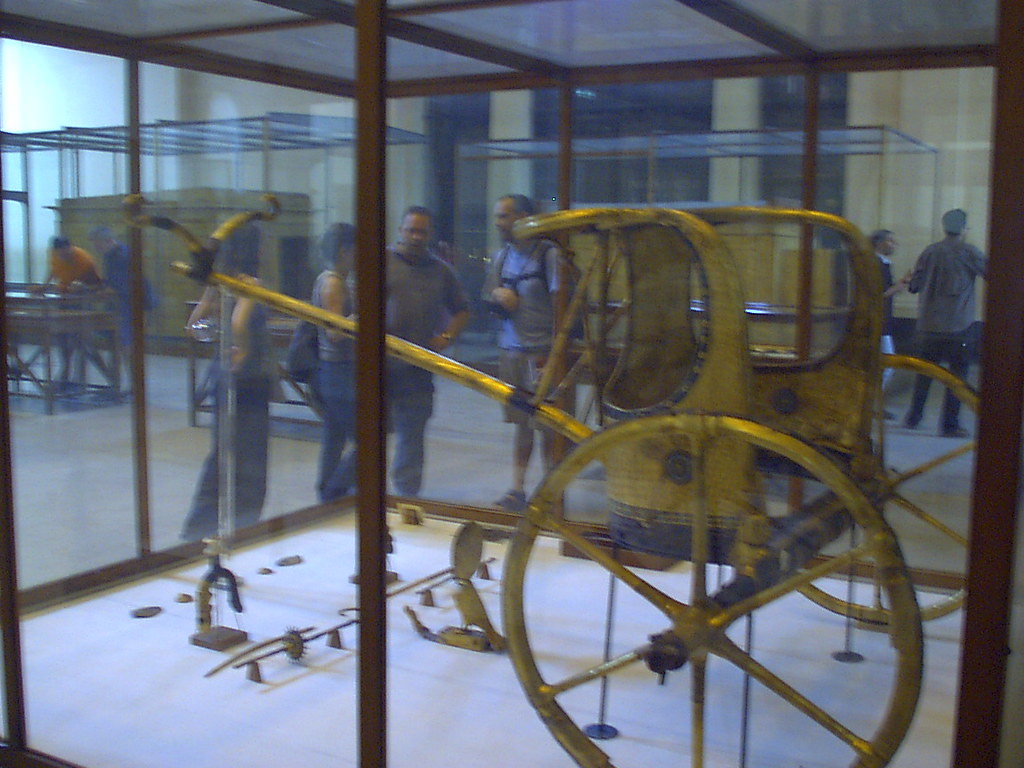This detailed color photograph captures an exhibition display inside a building. The primary focus is a display case made of glass and metal, containing a metal carriage with large spoked wheels. The body of the carriage is white, and it extends forward where one or two horses would be harnessed. Surrounding the carriage within the display case, additional objects are placed on the ground. Beyond the display case, several people are standing and conversing, while others are engaged with additional metal and glass display cases scattered throughout the background. The exhibition space is bustling with activity, as visitors explore and discuss the various exhibits.